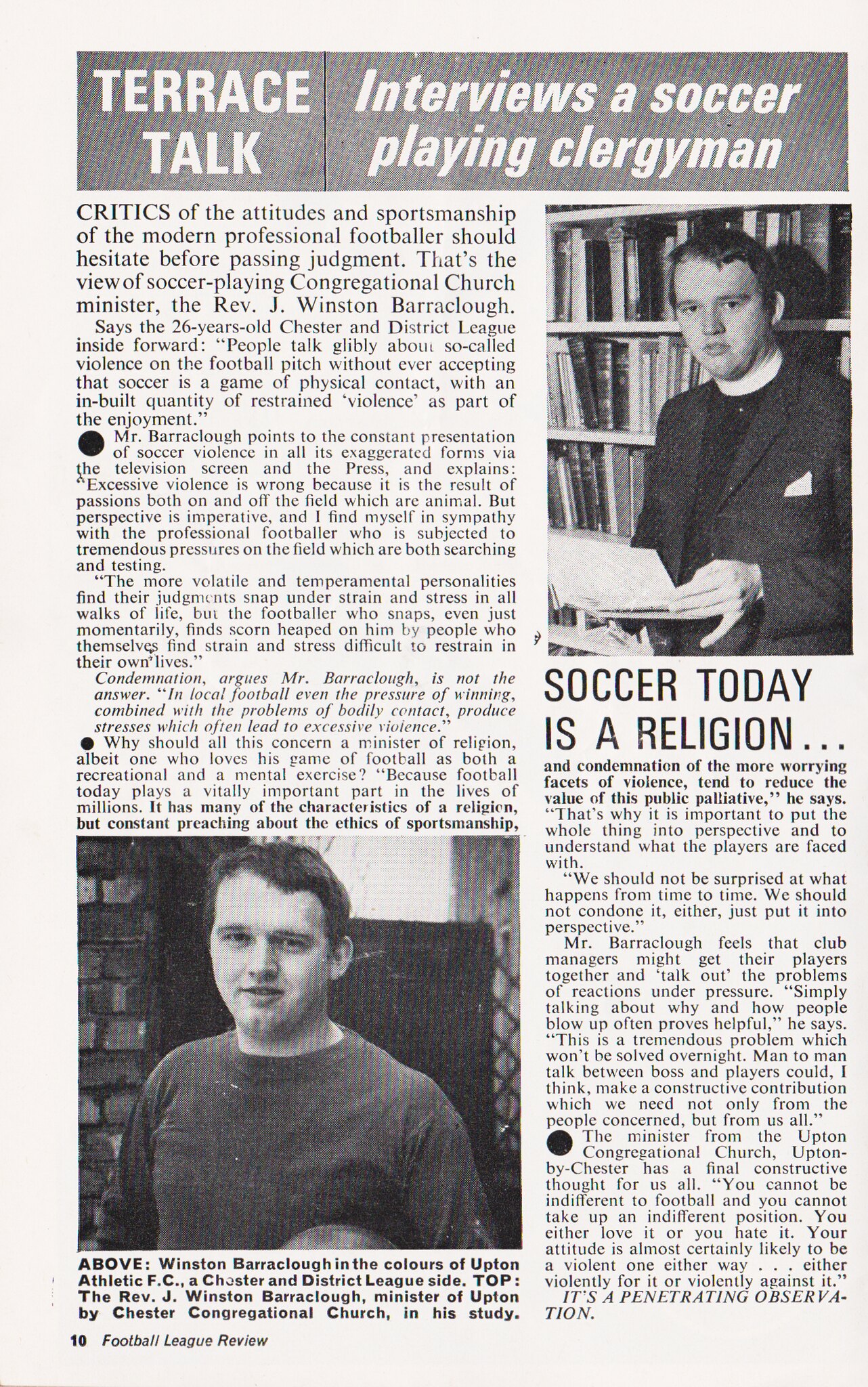The black and white page from the English football magazine features Terence Talk's interview with a soccer-playing clergyman. At the top, a gray-striped banner with bold white text reads, "TERENCE TALK on the left and "Interviews a Soccer Playing Clergyman" on the right. The page is divided into two main columns filled with small black text, describing an article that seems to include about seven paragraphs in total. 

At the top right, there's a photograph of the Reverend J. Winston Baraclough, Minister of Upton by Chester Congregational Church. He stands before a bookcase, wearing a black jacket with a white clerical collar and holding a book, probably a Bible, while looking at the camera. Below this image, a bold headline states, "Soccer Today is a Religion...”.

The bottom left of the page showcases another photograph of Reverend Baraclough, this time in a dark shirt, smiling while holding a football. He is identified in the caption as being featured with a ball for Winston Baraclough in the colors of Upton Athletic FC, the Chester and District League side.

At the bottom left in bold type, it reads, "Football League Review."

The overall layout effectively ties together the unusual intersection of faith and football in Reverend Baraclough's life, highlighting his dual roles as a clergyman and a passionate soccer player.